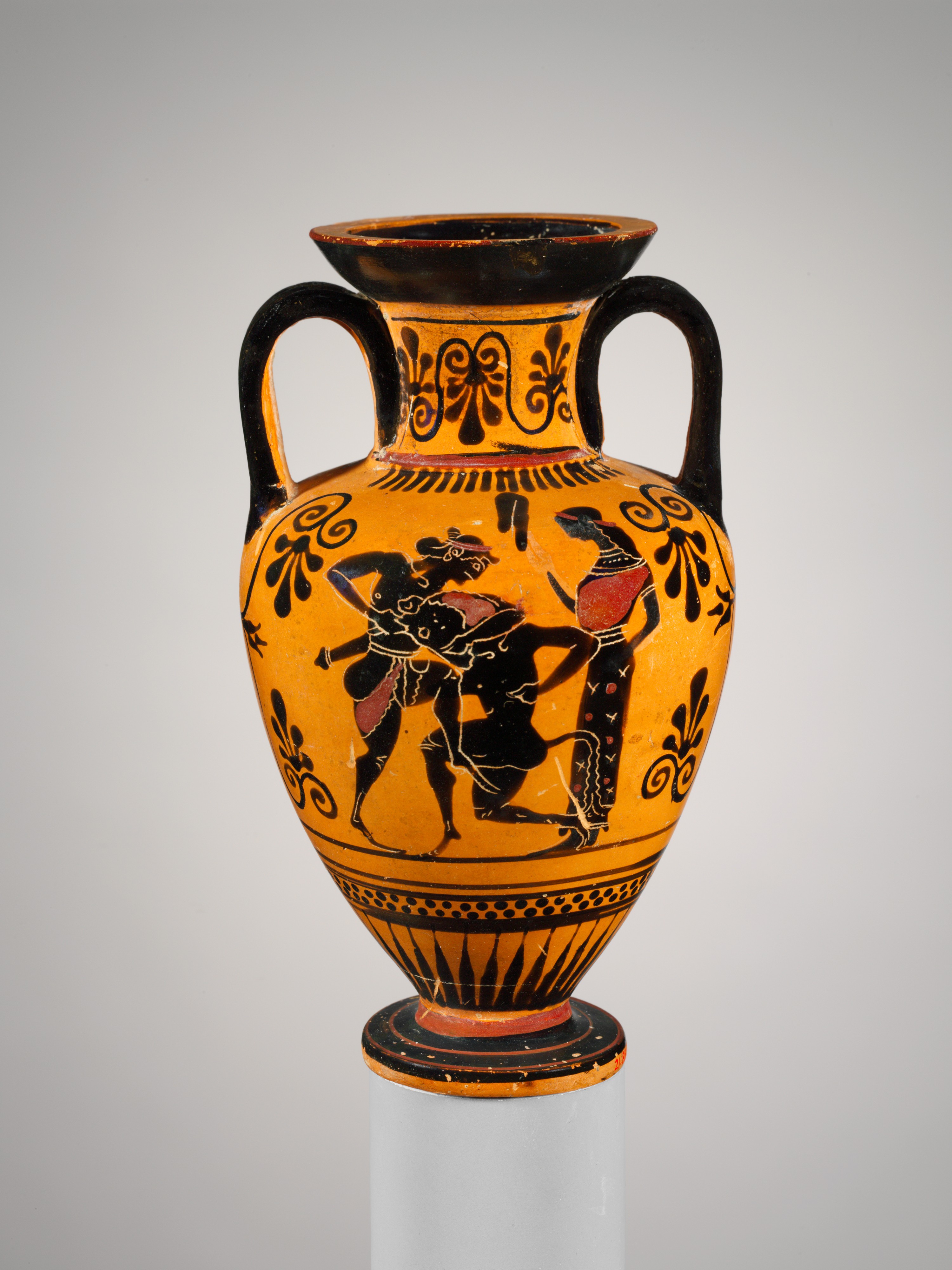This photograph features an ornate, ancient-looking vase, prominently displayed against a light gray background. The vase, which might be characterized as either an urn or a decorative container, is captured in portrait orientation and shows detailed craftsmanship indicative of either Greek or Egyptian artistry. 

The vase is primarily a vibrant yellow-orange with a brown rim at the top and features two large, black handles near the upper section. Each handle is detailed with yellow on the inside. The vase's wide body tapers to a narrower base decorated with intricate black patterns. These designs include checkered patterns, floral motifs, scrolling leaves, and arrows.

Central to the vase’s design are three silhouetted figures rendered in black. One figure kneels, seemingly engaged in a battle with another who stands with a raised leg. A third figure, a woman in a red toga-like shirt and a black patterned skirt possibly featuring birds and suns, stands behind them, holding a knife. The scene, interspersed with floral and geometric decorations, evokes an ancient narrative, perhaps from Greek or Egyptian mythology.

A black circular base supports the vase, and subtle shadowing beneath it hints at its solid presence on an unseen surface. The combination of vibrant colors, intricate patterns, and mythical imagery makes this vase a striking and historically rich artifact.